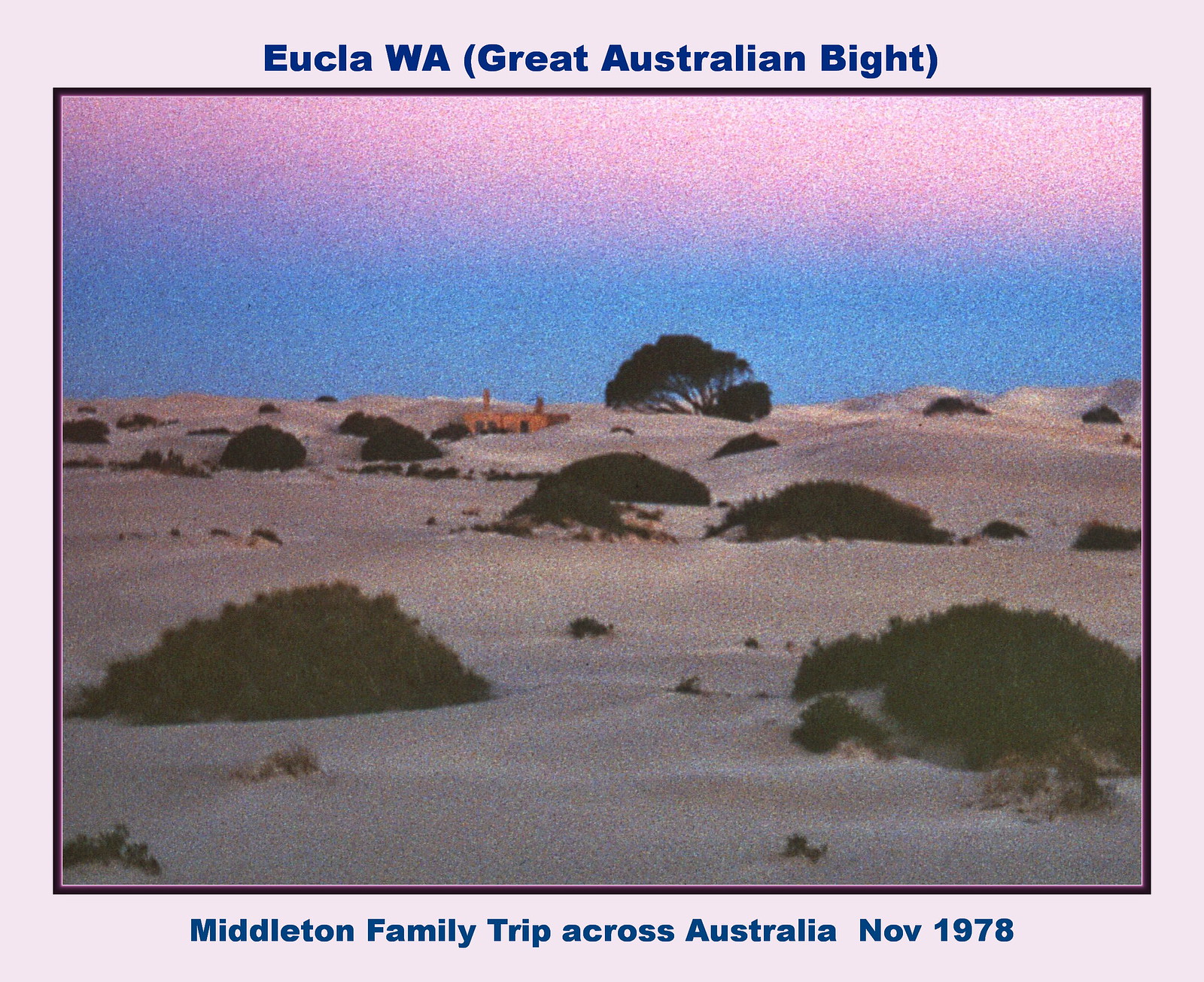The photograph, taken with an older, grainy camera in November 1978, shows a slightly blurry image of a landscape at dusk. It is bordered by a thin gray line and a heavier white border, suggesting it has been prepared for hanging. Across the top of the border, in distinctive blue text, is written "Eucla, WA, Great Australian Bight," and along the bottom in slightly lighter blue text, "Middleton Family Trip Across Australia, November 1978."

The scene captured in the photograph features a desert-like expanse with sandy hills and clusters of vegetation. The sky presents a gradient of colors transitioning from purplish-pink at the top to bluish-turquoise towards the horizon. The vast sandy landscape below includes large clumps of greenery such as kelp, low bushes, and a small tree near the horizon. To the left of the tree, there are two small brown structures that might be shacks or houses. In the central area of the image, closer to the water and amidst the sand, vague forms suggest the presence of people, perhaps on a towel, though the grainy quality makes this hard to confirm. This nostalgic and slightly ethereal snapshot perfectly captures the tranquility and vastness of the Great Australian Bight as experienced by the Middleton family on their cross-country journey.